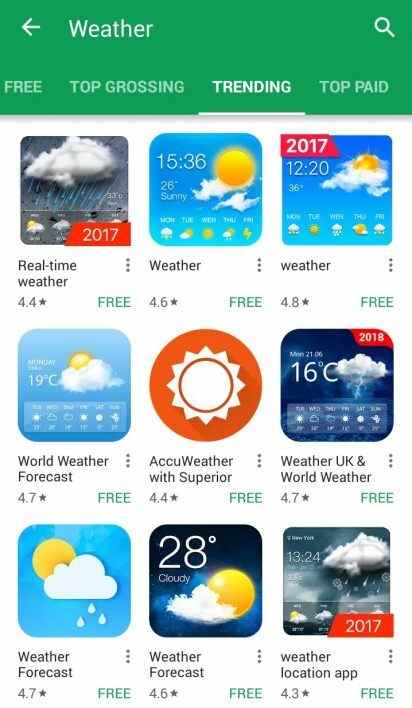This image illustrates a screenshot from an app store, showcasing the "Weather" category. At the top of the screen, a green banner spans the width, with a left-facing arrow icon on the left, labeled "Weather" in the center, and a search icon on the far right. Below the banner, navigation options for app categories appear, including "Free," "Top Grossing," "Trending," and "Top Paid," with "Trending" highlighted in white and underlined, indicating it is currently selected.

The main portion of the screen is dedicated to app icons displayed against a white background, organized in a grid consisting of three rows and three columns, totaling nine weather apps, all available for free:

1. **Top Left App:** "Real-Time Weather" – The app has garnered 4.4 stars and is marked as free.
   
2. **Middle Top App:** "Weather" – Featuring an icon depicting a weather screen, complete with time, sun surrounded by clouds, and a weekly forecast sample. It boasts 4.6 stars and is listed as free in the bottom right corner.

3. **Top Right App:** "weather" – Displayed in lowercase, the icon mirrors the previous app's design and includes a banner indicating the year "2017". It has achieved a rating of 4.8 stars and is free.

Below these, the next two rows continue the listing of weather apps, each similarly styled and categorized, yet their detailed descriptions are not provided in the aforementioned text.